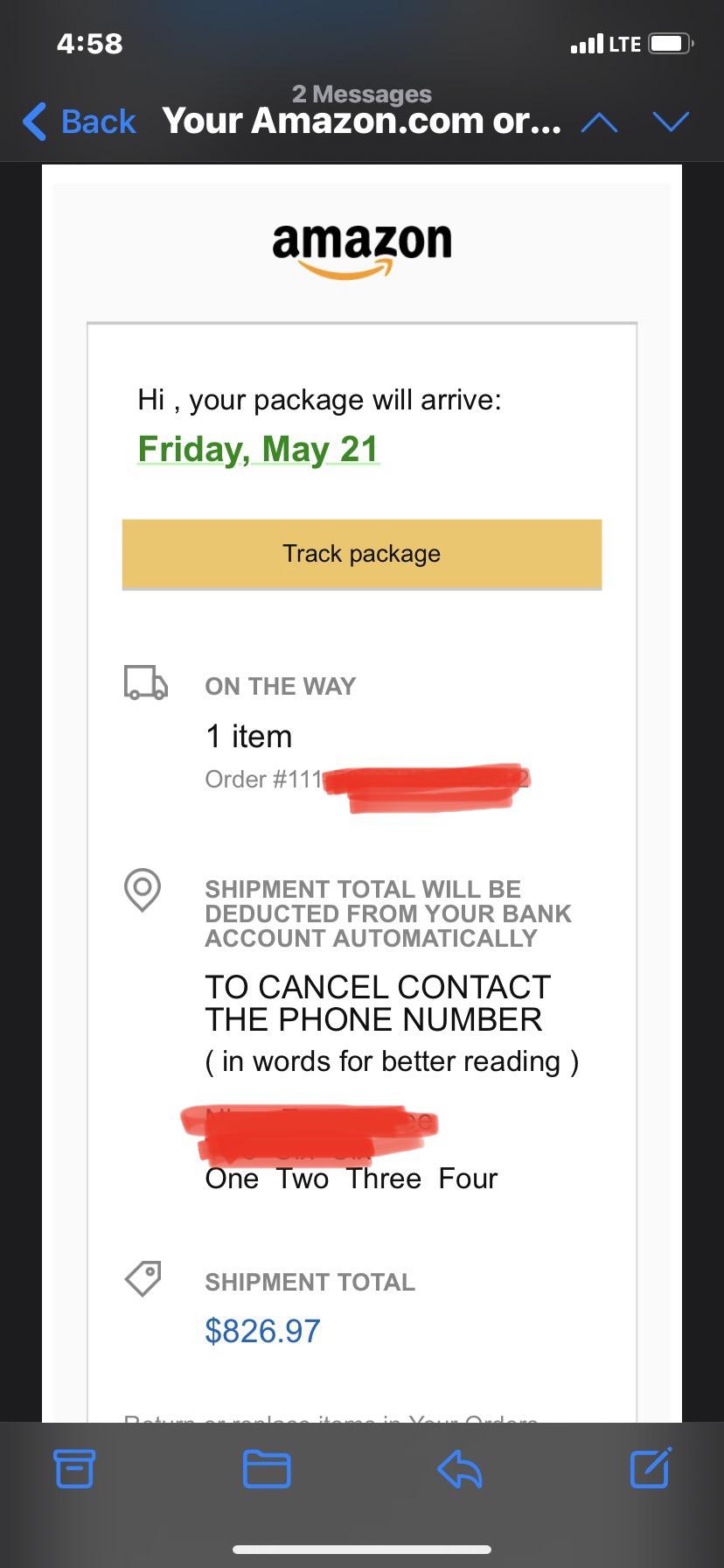The image features a smartphone screenshot against a black background, located at the top left corner. The phone's screen shows the time as 4:58, four signal bars, and a battery status that is approximately four-fifths full. Below this are notifications indicating "2 messages."

A blue arrow pointing left is labeled "Back," and beneath this is text in white reading "Your Amazon.com or..." accompanied by up and down arrows. Below this upper section, a light gray box displays the Amazon logo at the top. The text within this box reads: "Hi, your package will arrive Friday, May 21st."

An orange box follows underneath, prompting with "Track Package." Below the orange box, there is an image of a delivery truck with accompanying text: "On the way: 1 item. Order number," with the specific order number redacted. Further down, it mentions, "Shipment total will be deducted from your bank account automatically."

In bold letters, it states: "To cancel, contact," followed by a phone number, which is redacted in red for privacy. More down the message, specific details concerning the shipment total ($826.97) have also been partially obscured in red.